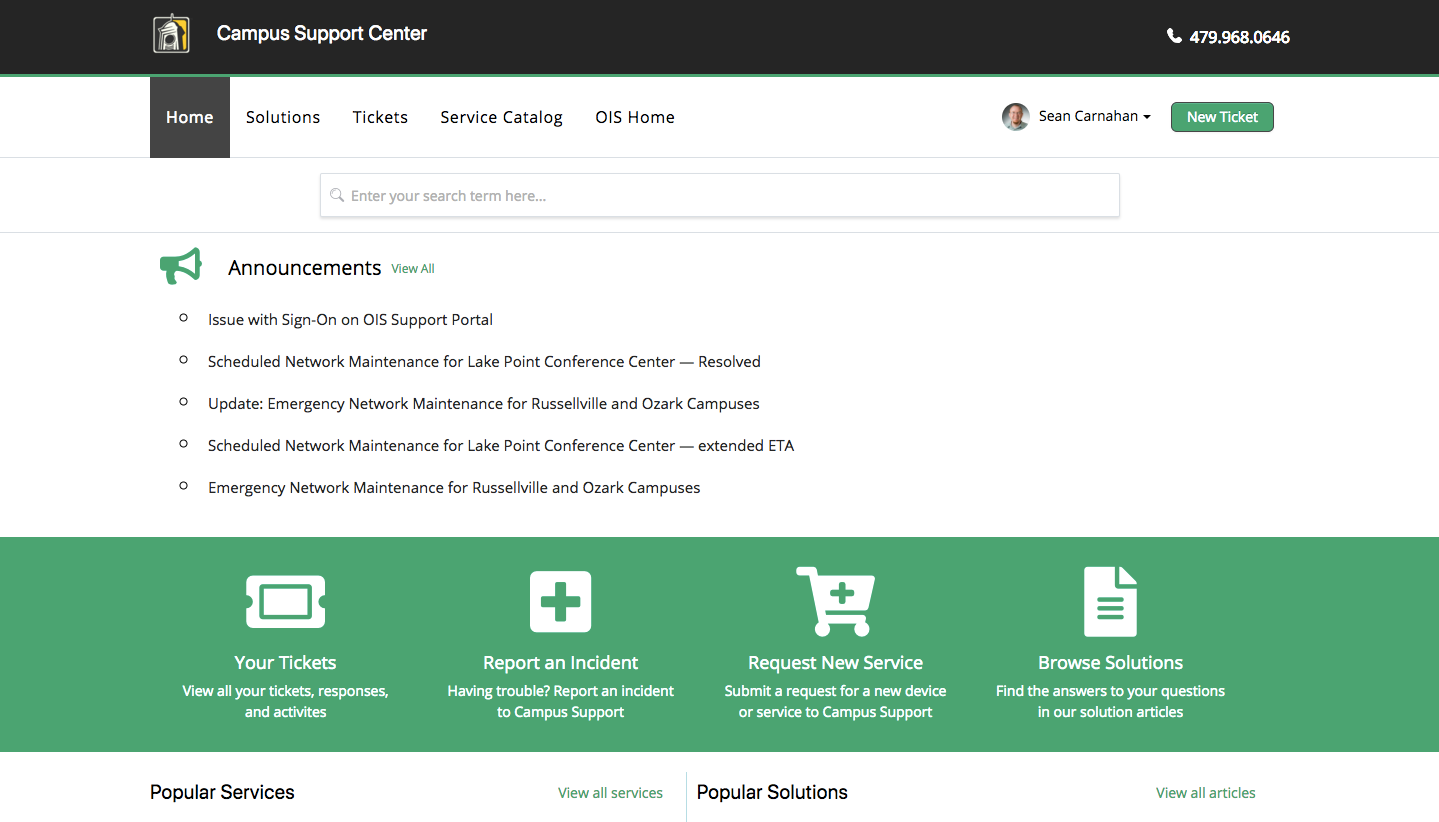The image features a user interface on a white background. At the top, there is a black header labeled "Campus Support Center," which includes a small silver square resembling a doorknob. Adjacent to this, on the right side, is an icon of a phone with the number "479-968-0646."

Below the header, the white background continues, framing a smaller black square that encircles various navigation options: "Home," "Solutions," "Tickets," "Service Catalog," and "DIS Home." Further down, a circular icon displays a picture of Shawn Carnahan, with a dropdown arrow beside his name. 

To the right of Shawn Carnahan's image, there is a prominent green button labeled "New Ticket." Beneath this section, a long search box is positioned for user input. Below the search box, a green horn icon leads to announcements, with a link to "View All." The following announcement texts appear:

- "Issue with sign-on DIS support"
- "Scheduled Network Maintenance for Lake Point Conference Center resolved"
- "Update: Emergency Network Maintenance for Russellville and Ozark Campuses"
- "Scheduled Network Maintenance for Lake Point Conference Center extended ETA"
- "Emergency Network Maintenance for Russellville and Ozark Campuses"

Each announcement is accompanied by a small circle.

Lastly, a large green box with the title "Your Tickets" in white text offers links to "Report an Accident," "Request New Service," or "Browse Solutions." Beneath this section, the interface on a white background highlights links to "Popular Services," "View All Services," "Popular Solutions," and "View All Articles."